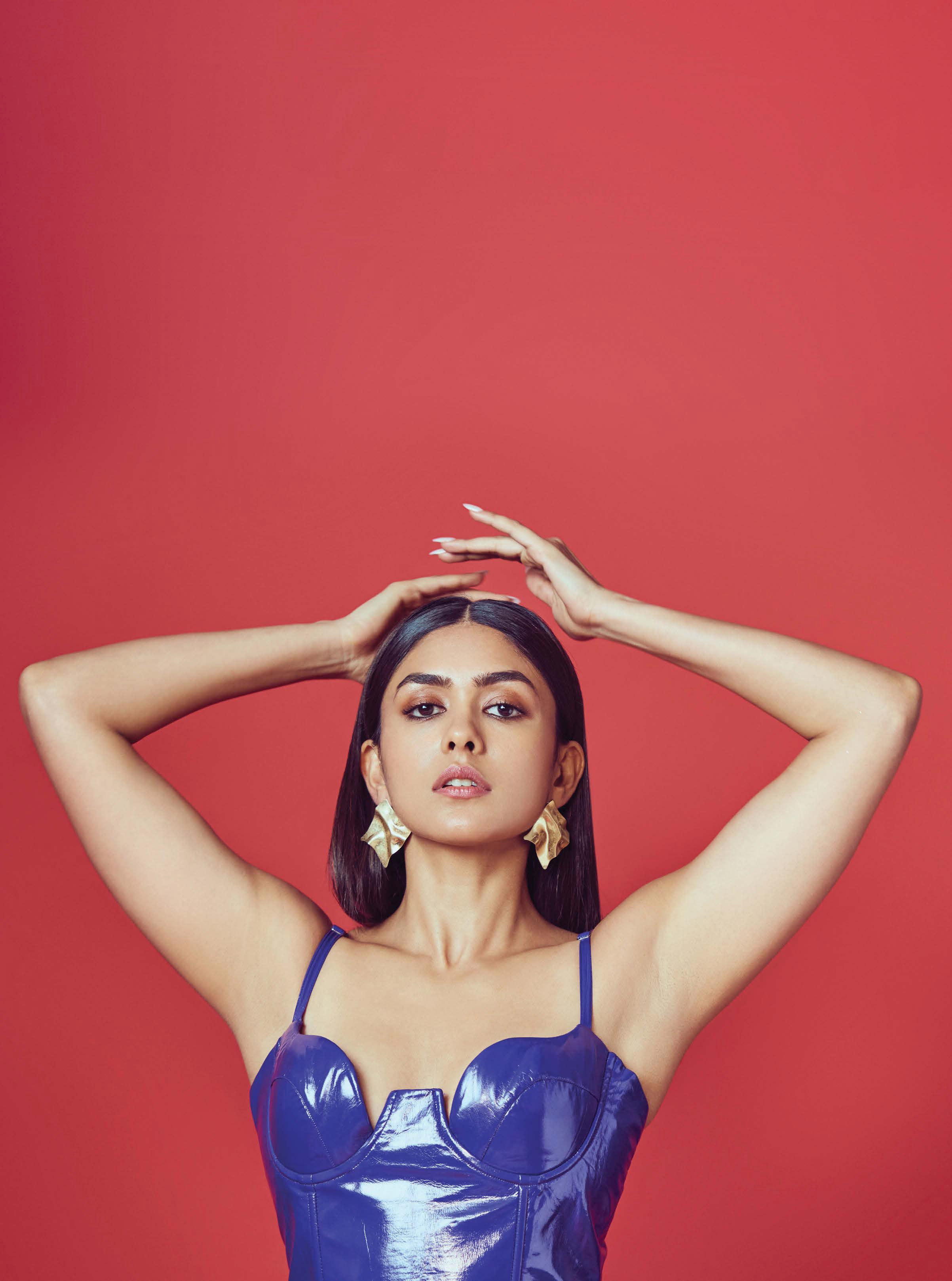This photograph captures a woman elegantly posing against a rich reddish-pink backdrop that spans the entire frame. The woman is centrally placed, with the composition showing her from just above the waist to the top half of the image. She has striking long black hair that cascades down her back, framing her face adorned with bushy eyebrows and expressive brown eyes. Her gaze is direct, engaging the camera, while her pink full lips are slightly parted, revealing a hint of her white front teeth.

Adding to her sophisticated look, she wears large, square gold earrings that accentuate her features. Her attire is a sleeveless, purplish dress with a shiny texture and two delicate straps, reflecting a bit of light in the center from her chest downward. 

Her left arm is raised, bending at the elbow with fingers extended and poised gracefully about an inch above her head. Her right arm stretches upward then bends at the elbow; the fingers of her right hand are artfully placed behind her head, leaving just her pinky and ring fingers visible atop her head. This intricate pose, combined with her expressive features and stylish outfit, creates a captivating and refined image.